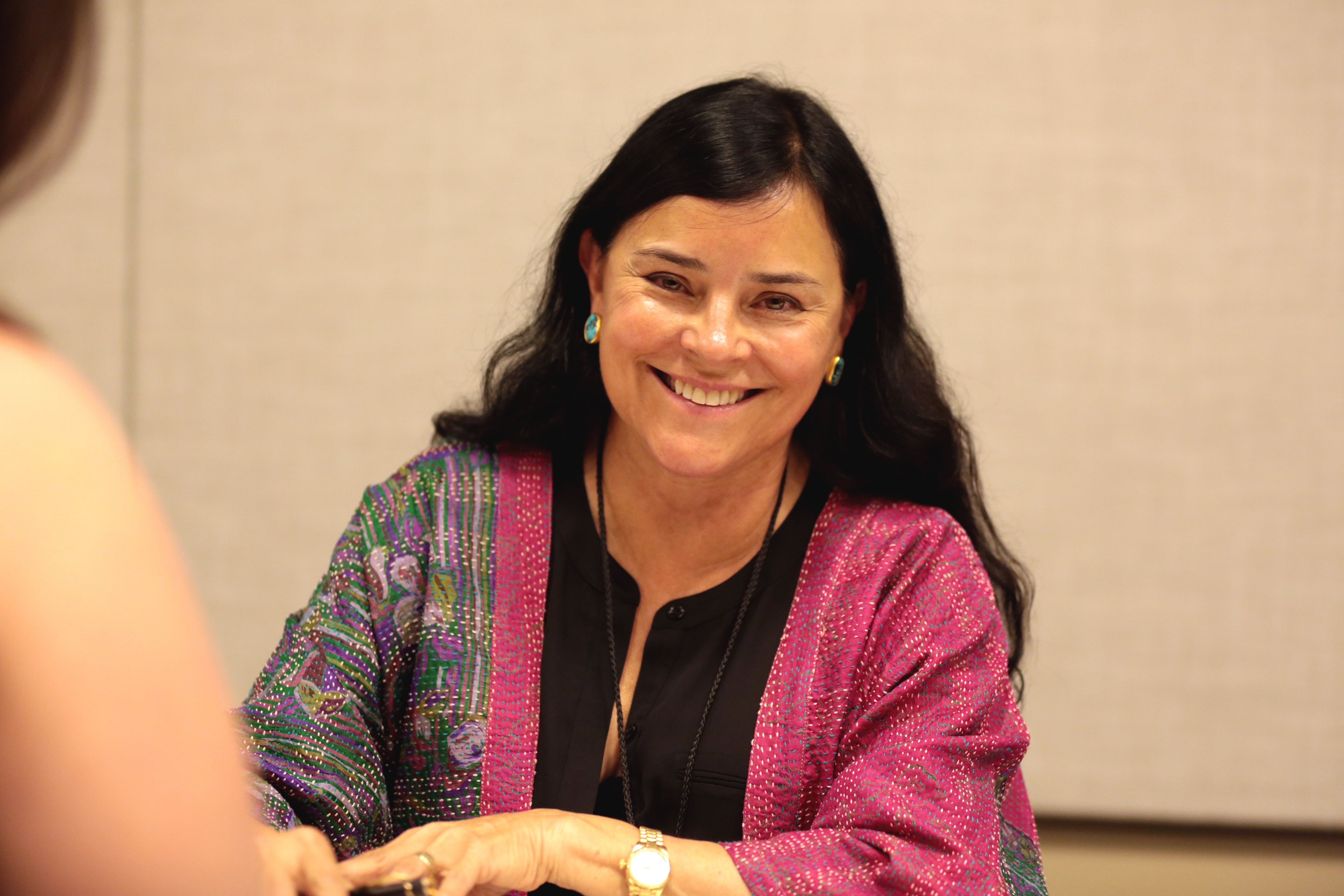The photograph captures a cheerful older Caucasian woman, likely in her 50s or 60s, with long black hair, sitting in what appears to be a conference room or gymnasium. She is smiling warmly, exuding a friendly and approachable demeanor. She is dressed in a distinctive top coat that is solid pink on one side and a vibrant plaid pattern of purple, green, and blue on the other. Beneath the coat, she wears a black top with a button undone at the collar, revealing a black necklace that extends below her chest. Her left wrist is adorned with a gold wristwatch, and a gold ring decorates her ring finger. Large green circular earrings dangle from her ears, completing her ensemble. 

In the background, a grey fabric panel wall adds a neutral tone to the setting, while the partial view of another woman's hair and shoulder on the left edge of the frame adds a layer of context to the environment. The older woman’s overall appearance, her vibrant attire with a touch of sparkle, and her joyful expression create a captivating and detailed portrait.